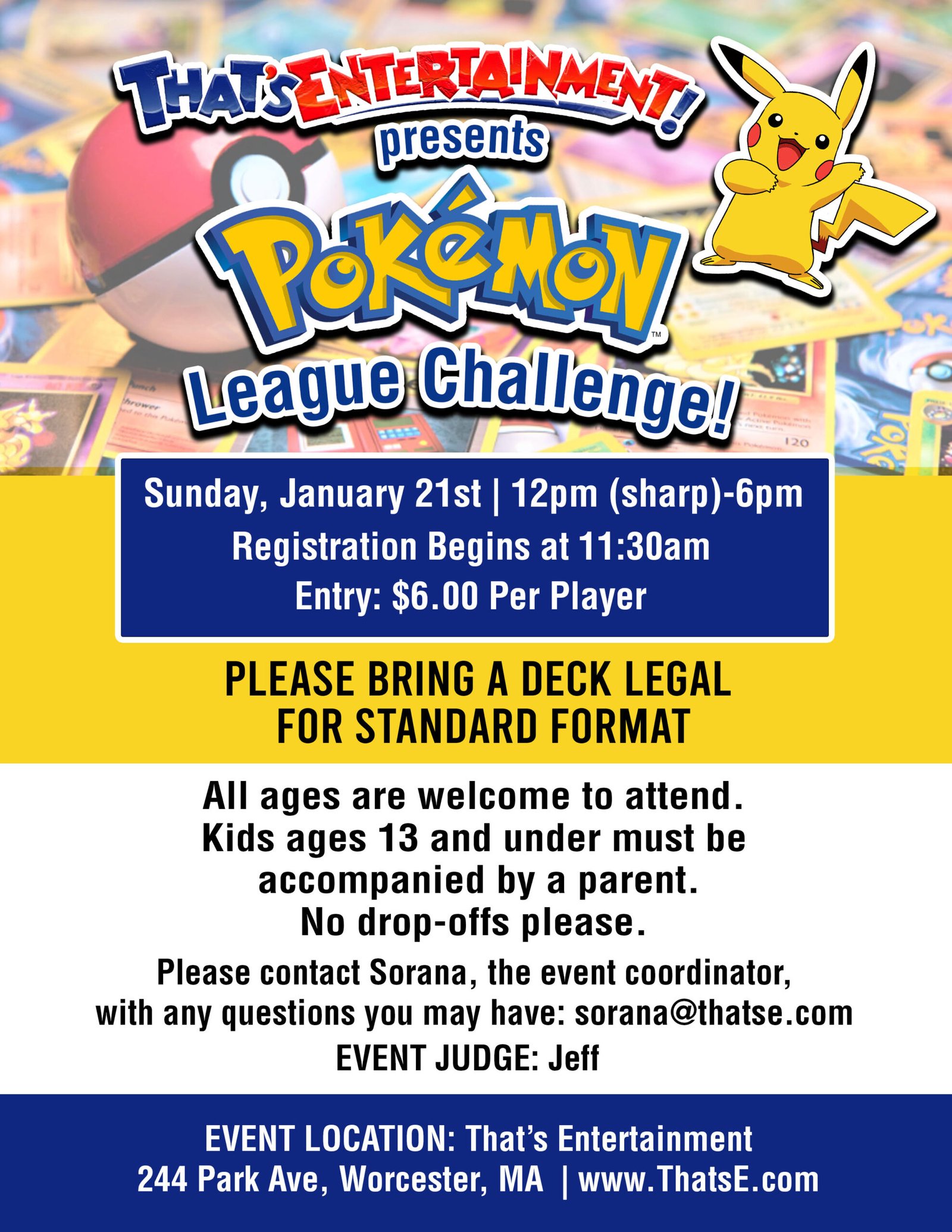**Poster Description for Pokémon League Challenge Event**

The poster for the Pokémon franchise features vibrant and engaging imagery centered around a prominent Pokémon character, with an array of Pokémon cards showcased in the background. At the top, the text boldly reads, "That's Entertainment! presents Pokémon League Challenge!" capturing attention with enthusiastic exclamations.

A striking blue banner runs through the middle of the poster, providing key event details: 
- **Date and Time:** Sunday, January 21st, from 12 p.m. sharp to 6 p.m.
- **Registration:** Begins at 11:30 a.m.
- **Entry Fee:** $6 per player.

Beneath the banner, a distinct yellow box highlights an important note: "Please bring a deck legal for standard format."

In a white section with black text, further event information is provided:
- **All Ages Welcome:** Children aged 13 and under must be accompanied by a parent. No drop-offs, please.
- **Contact Information:** For questions, attendees can reach out to Saranya, the event coordinator, at saranya@thatse.com.
- **Event Judge:** Jeff will oversee the event.

Finally, the poster’s bottom edge features a blue border with white text, giving the event location details:
- **Location:** That’s Entertainment, 244 Park Avenue, Worcester, Massachusetts.
- **Website:** www.thatse.com.

This is a call-out for the Pokémon League Challenge, ensuring that all necessary information is clearly communicated for interested participants. Don’t miss this exciting event organized by That's Entertainment!